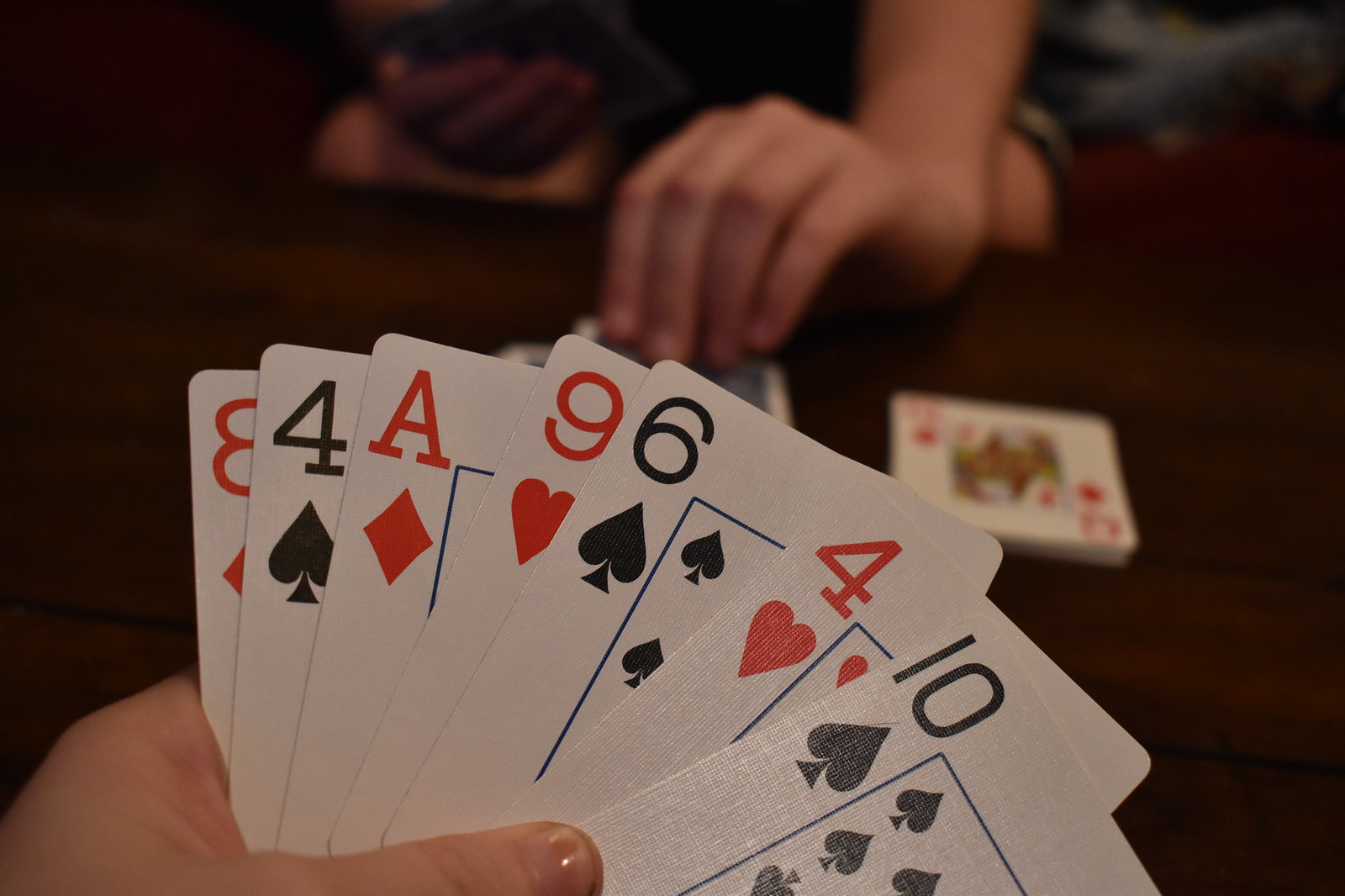In this detailed image, an individual is prominently displaying a fan of playing cards in their hand. The cards revealed include the 8 of Diamonds, 4 of Clubs, Ace of Diamonds, 9 of Hearts, 6 of Clubs, 4 of Hearts, and 10 of Clubs. Across from this person is another individual, though their cards are obscured from view as they hold them privately. This second person appears to be in the process of drawing a card from a faced-up card stack placed at the center of the brown table between them. Adjacent to the faced-up stack is a facedown card, which is discernible as a Queen, likely either of Diamonds or Hearts, though it's not clear which. The scene is slightly blurred around the second individual, though you can make out their lower body attire, likely shorts, and their kneecaps. The color of the cards is true to their traditional suits, with red cards appearing red and black cards appearing black.